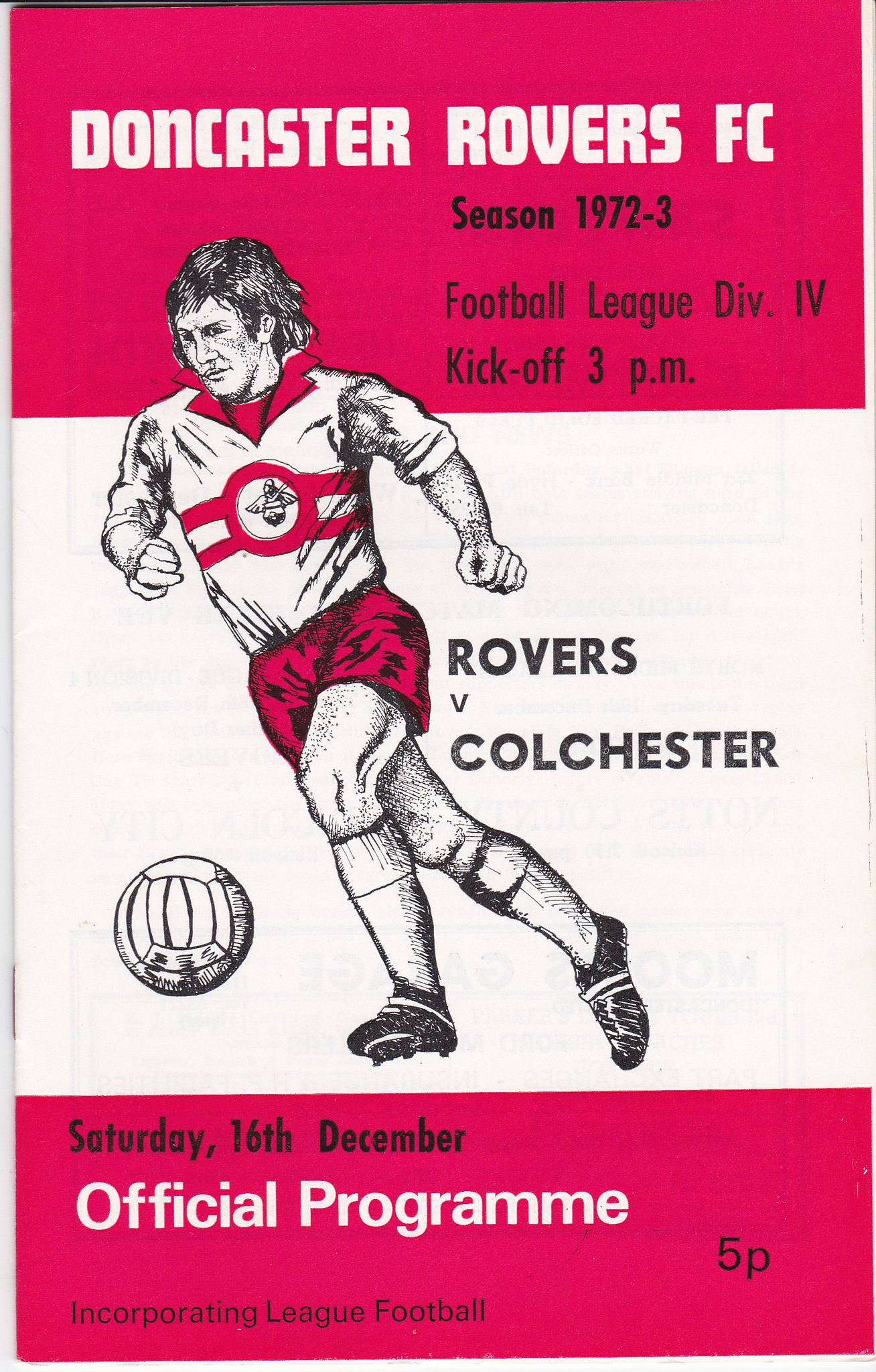The image is a photograph of the cover of a program for an English football match. The cover predominantly features red, white, and black colors. At the top, against a red background, white text reads "Doncaster Rovers FC". Directly below, in black letters, it states "Season 1972-3" and then "Football League Division IV" (in Roman numerals) followed by "Kickoff 3 p.m." The central part of the cover showcases an illustration of a soccer player. The player is centered on a white background, depicted in mid-run and either kicking or about to kick a white soccer ball positioned near his feet. He is dressed in a white jersey with a red collar, a red circle in the middle, two horizontal red stripes extending from the circle, red shorts, white socks, and black cleats. To the right of the player, black text reads "Rovers vs. Colchester." Below this, against a red background, black text indicates "Saturday 16th December," and further down, it reads "Official Program." Additionally, at the bottom left in black text is "Incorporating League Football," and at the bottom right, "5P" in black letters.